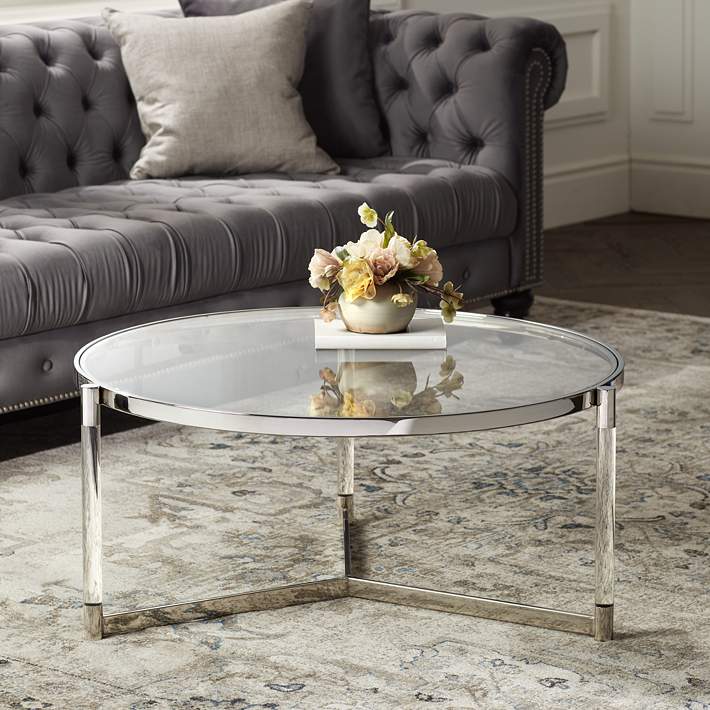In a stylish, modern living room, a circular glass coffee table with a silver trim and uniquely designed see-through legs stands prominently. On the table, a book and a vase filled with several dead flowers capture attention. The table is set on a large white carpet adorned with intricate gray and floral patterns. To the left, a sophisticated tufted gray sofa, likely upholstered in fabric, features a mix of light and deep gray throw pillows that enhance its elegant appearance. The space rests on a dark brown wooden floor, with off-white walls serving as the backdrop, creating a cozy yet contemporary ambiance. This detailed setup, with its carefully chosen monochromatic palette, exhibits a tasteful blend of aesthetics and comfort, indicative of professional home design.